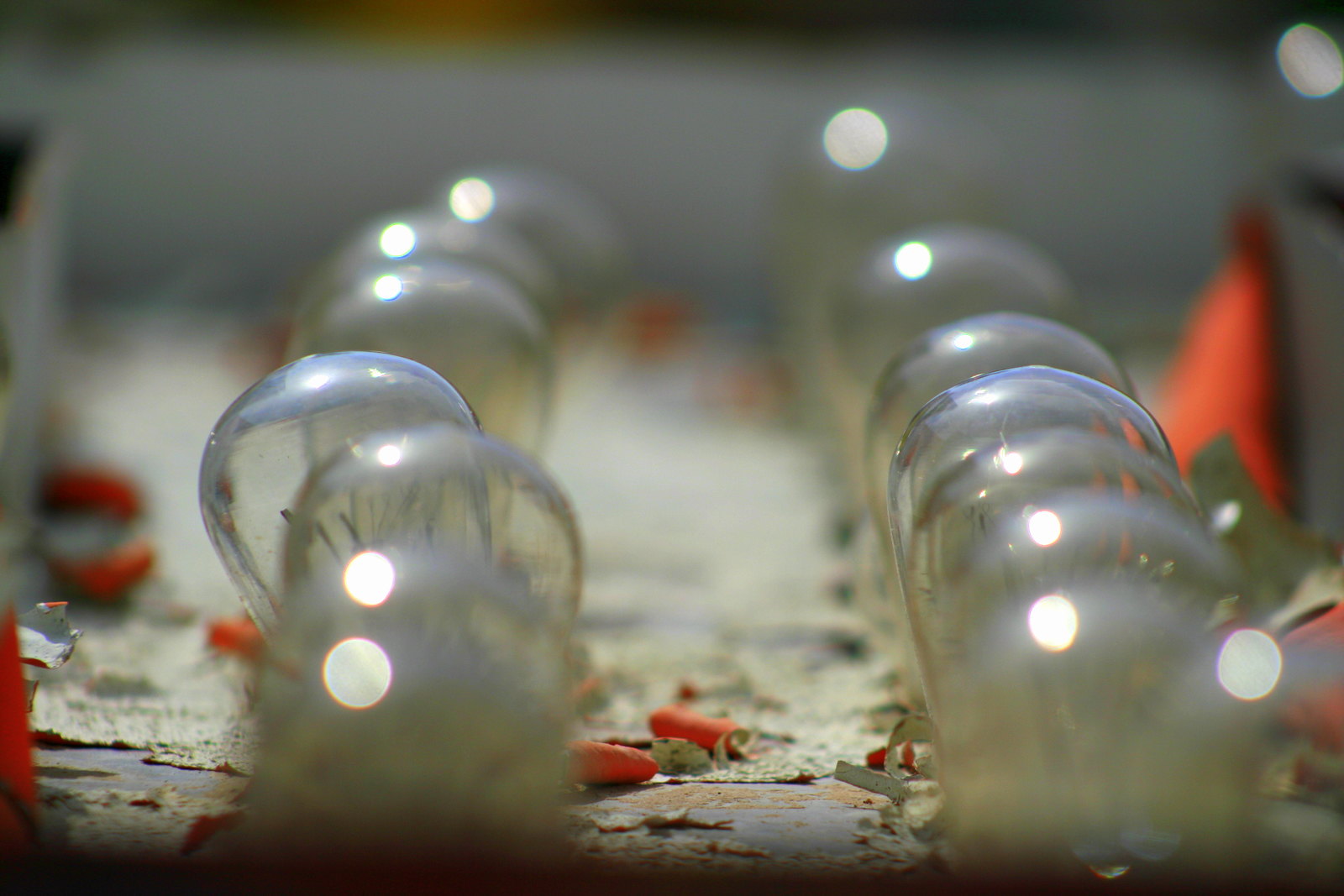This photograph captures a close-up view of approximately 10 to 12 clear, unlit light bulbs arranged in two parallel rows. The bulbs appear to be part of a sign or installation. The focus of the image is sharper in the middle, while the bulbs in the foreground and background are blurred. The surface beneath the bulbs is worn and textured, revealing peeling paint in shades of red and orange atop a rusty, off-white metal base. Debris and fragments of peeling paint scatter around the bulbs, adding to the image's gritty, industrial aesthetic. There are no people or text in the photograph, and the setting appears to be indoors, with ambient light creating a soft glare on some of the bulbs.